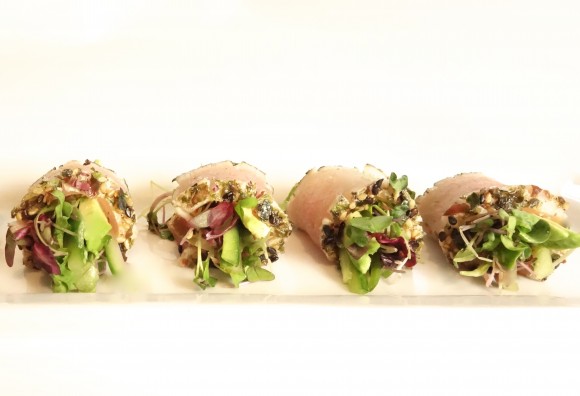The image features four robust salad wraps, positioned side by side from the lower left to the lower right of the frame. Each wrap is encased in a light tan tortilla that fully encloses their vibrant fillings. The wraps are generously stuffed with an assortment of fresh vegetables, including crisp lettuce, creamy avocado slices, and possibly some green peppers or cucumbers. A mixture that resembles a seed spread adds texture to the filling. The background is a bright white surface, likely a light cream-colored counter, which contrasts with the wraps and ensures the colorful ingredients are prominently displayed. The ends of the wraps are open, facing the camera, showcasing their plentiful and appetizing contents.